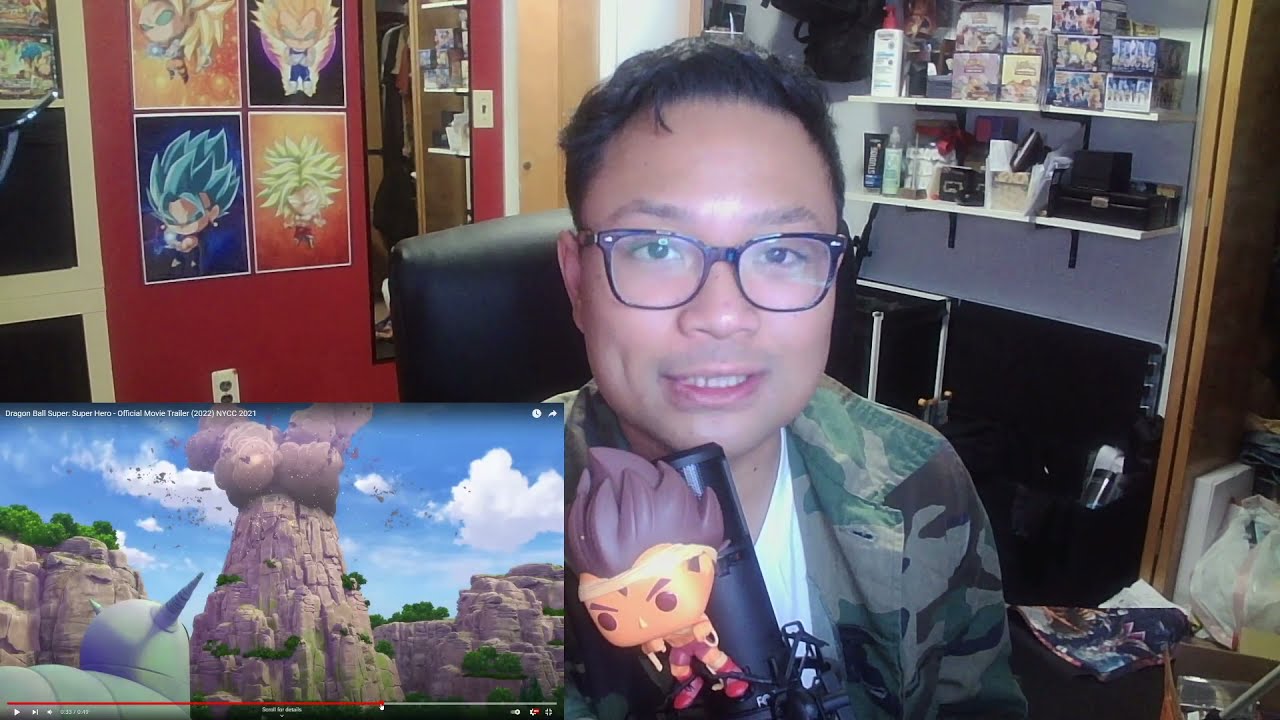A detailed image shows an Asian man with short black hair and black-framed glasses, live streaming a video game, likely on YouTube, from his gaming room. He is seated at a desk, wearing a camo print shirt or jacket with a white undershirt. In front of him is a long black microphone adorned with a Funko Pop figure. A screen capture of the YouTube video he's sharing is visible in the bottom left corner of the image, depicting a game with mountains, sky, and clouds. The backdrop of his room reveals a red wall decorated with Dragon Ball Z and other anime posters, indicating his ardor for anime. Shelves filled with various anime toys and other collectibles, including boxes of Pokemon cards, further illustrate his passion for "nerdy" interests and complete the scene of an enthusiastic gamer and anime fan engaging with his online audience.